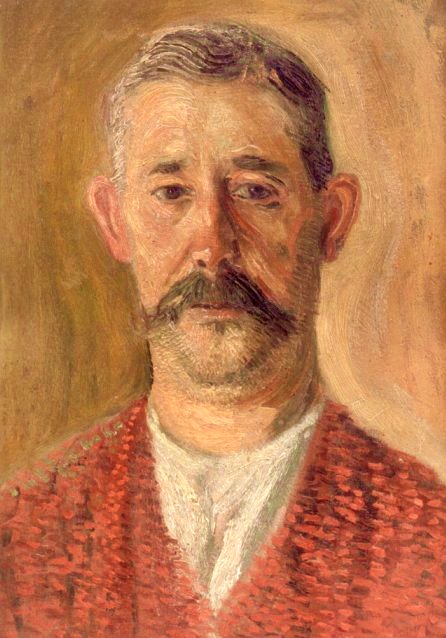This image features a detailed portrait painting of a man, primarily focusing on his face and upper body. The man has short, light brown hair with hints of gray, thin eyebrows, and sideward-looking eyes that convey a sense of sadness or nervousness. His facial hair includes a large, black mustache and some gray stubble on his chin, adding to the aged appearance marked by visible wrinkles. 

He is dressed in a white t-shirt underneath a red jersey or sweater. The background, which appears brown with greenish undertones and a wavy shape, creates a simple yet classical ambiance, likely painted using oil techniques. This portrait, with its detailed rendering and emotional depth, suggests a blend of country western elements and traditional aesthetic styles.